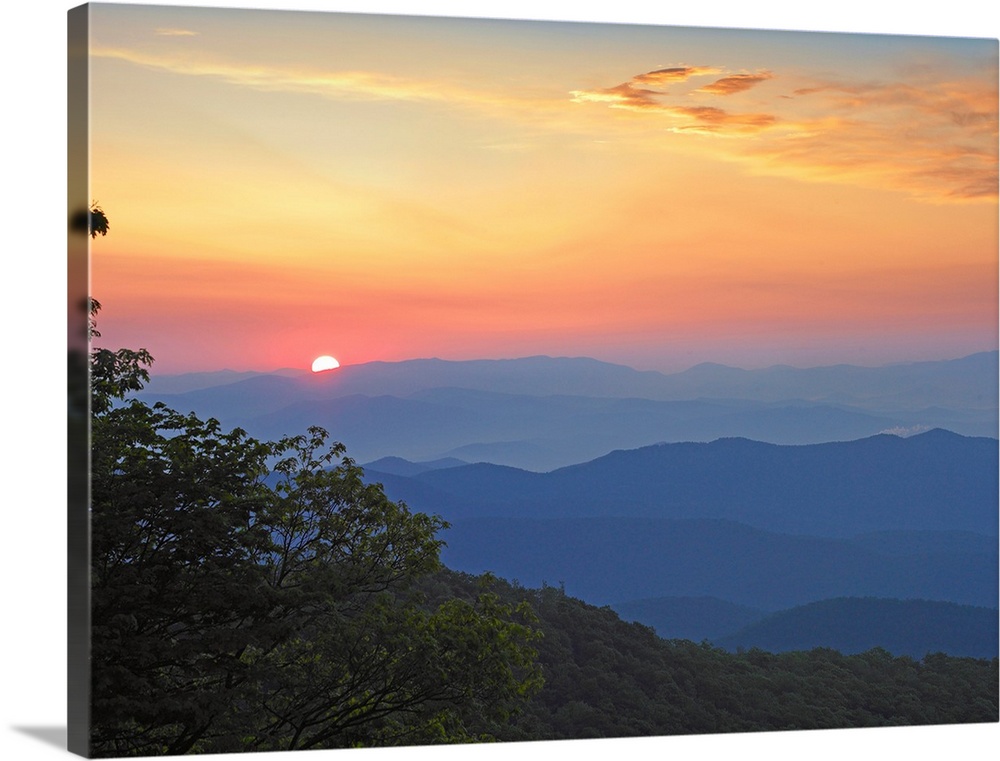This image showcases a breathtaking nature scene, likely captured in Hawaii, presented as a high-quality canvas print. The foreground of the image features the lush, green canopy of a dense forest, with an array of vibrant tree leaves and shrubbery. On the bottom left corner, there's a detailed close-up of a green-leafed tree. The viewer’s perspective appears to be from atop a mountain, looking down over verdant hills that eventually lead to a distant mountain range.

The mountains in the background transition from green to a serene blue, enveloped by a misty fog that enhances their majestic appearance. The horizon is graced by a stunning sunset, with the sun itself just barely peeking out from behind the mountain range. This creates a mesmerizing gradient in the sky, blending shades of golden yellow, orange, peach, and purple, with hints of blue interspersed. The sunset's warm hues reflect beautifully onto the scattered clouds, adding depth and splendor to the scene.

Overall, this beautifully composed image blends vibrant foreground details with a serene, colorful sunset, making it an exquisite representation of nature's beauty on canvas.